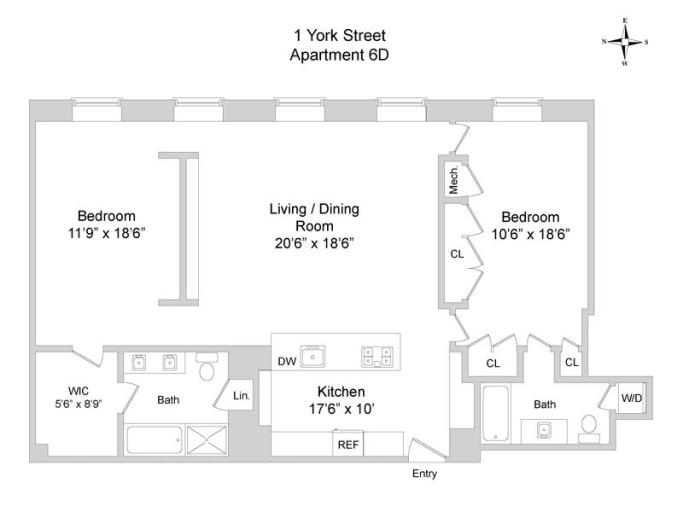**Detailed Floor Plan of Apartment 6D at One York Street**

This detailed floor plan showcases a two-bedroom, two-bathroom apartment located at One York Street, Apartment 6D. 

- **Entryway:** The apartment entry is located at the bottom right side of the plan, clearly marked with the word "ENTRY." 
- **Living and Dining Area:** Centrally situated, the living/dining room measures a spacious 20' 6" x 18' 6", providing ample space for both relaxation and dining.
- **Bedrooms:** 
    - **Master Bedroom (Upper Left):** This room measures 11' 5" x 18' 6", offering a comfortable and roomy space.
    - **Second Bedroom (Right):** This bedroom is also well-sized, situated adjacent to the second bathroom.
- **Kitchen:** The kitchen occupies the lower center of the plan, designed as a walk-in or galley kitchen with dimensions of 17' 6" x 10'. This efficient layout provides plenty of counter space and storage.
- **Bathrooms:** 
    - **Bathroom (Lower Left):** Adjacent to the walk-in closet (WIC) and a linen closet, this bathroom is conveniently located next to the master bedroom.
    - **Second Bathroom (Lower Right):** Positioned close to the second bedroom, this bathroom offers easy accessibility.
- **Additional Features:** A walk-in closet (WIC) is situated in the lower left corner, providing additional storage space.

The floor plan includes a small compass in the upper right corner indicating that north is to the left, east is at the top, south is to the right, and west is at the bottom, aiding in spatial orientation.

Each room is labeled with its specific dimensions, ensuring a precise understanding of the space. Notable dimensions include:
- Master Bedroom: 11' 5" x 18' 6"
- Living/Dining Room: 20' 6" x 18' 6"
- Kitchen: 17' 6" x 10'
- Second Bathroom: 10' 6" x 18'

This floor plan provides a comprehensive and detailed view of Apartment 6D at One York Street, giving potential residents a clear idea of the layout and space distribution.